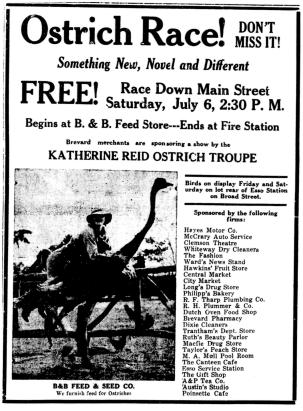This black-and-white photo depicts a detailed outdoor sign advertising an upcoming Ostrich Race, promising an exciting and unique event that the public shouldn't miss. The sign, full of engaging details, reads: "Ostrich Races - Don't Miss It! Something New, Novel, and Different, Free!" The race is scheduled to take place on Main Street on Saturday, July 6th, at 2:30 PM, starting at B&B Feed Store and concluding at the Fire Station. Sponsored by Brevard Merchants, the event features a special show by the Catherine Reed Ostrich Troupe. Additionally, the troupe's birds will be on display on Friday and Saturday at the lot behind East Station on Broad Street. 

The numerous local sponsors include Helen Hayen Motor Company, McCrary Auto Service, Clemson Theater, Whiteway Dry Cleaners, The Fashion, Ward's Newsstand, Hawkins Fruit Store, Central Market, City Market, Long's Drug Store, Phillips Bakery, R.F. Tharp Plumbing Company, R.H. Plumber & Company, Dutch Oven Food Shop, Brevard Pharmacy, Dixie Cleaners, Trantham's Department Store, Roth's Beauty Parlor, Mace McPhee Drug Store, Taylor's Peach Store, M.A. Mel Pool Room, The Canteen Cafe, S.O. Service Station, The Gift Shop, A&P Tea Company, Austin Studio, and Poissonette Cafe. 

A grainy photograph within the advertisement captures a person, possibly a woman, riding an ostrich, accentuating the exotic and entertaining nature of the event.